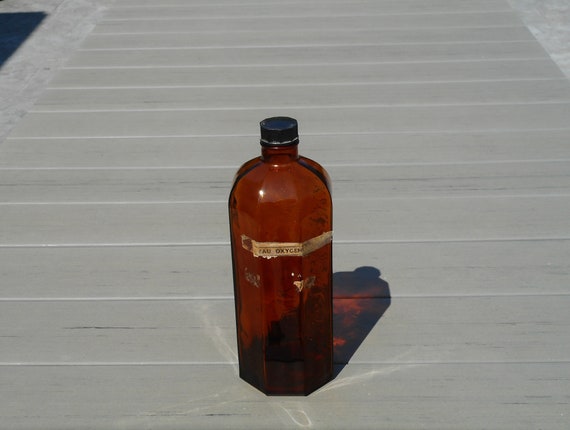The image features an antique-style bottle situated on a light gray, slatted wooden platform, resembling a clean dock. The wooden slats are horizontally aligned, with visible grain adding texture to the scene. The bottle, composed of dark reddish-brown glass, has a historical pharmacy aesthetic with a beveled cylindrical shape and a subtle base that may be hexagonal or pentagonal, tapering to a rounded mouth. It is capped with a black lid, possibly made of metal or plastic. A tattered, off-white label with the remnants of text, including partially legible words like "oxygen" or "oxy-sem," is affixed across the front with brown tape. A small amount of liquid is visible at the bottom of the bottle, which casts a shadow to the right, enhancing the depth of the scene. In the top left corner, a glimpse of water framed by the dock adds a subtle hint of context to the outdoor setting.